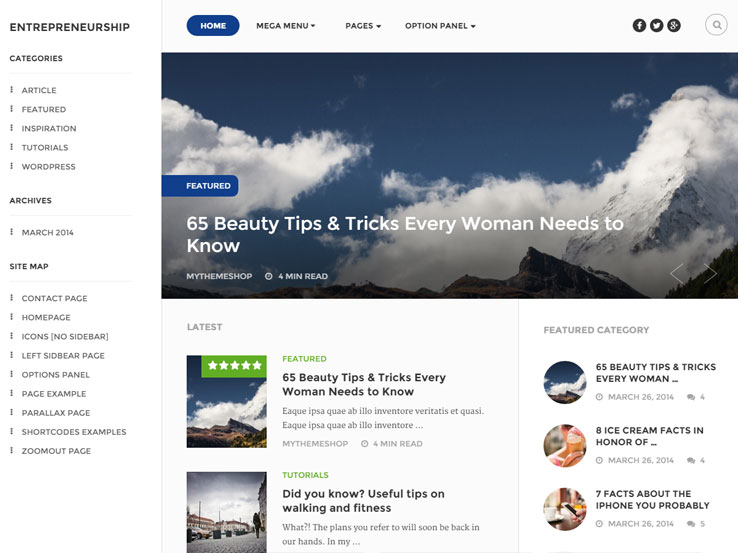In the advertisement for entrepreneurship seen online, the layout is structured with a variety of navigational and informational elements. On the far left, the word "Entrepreneurship" is prominently displayed as the main header. Moving right across the top, there are menu options labeled "Home," "Mega Menu," "Pages," and "Option Panel." Further to the right on the same line, three icons represent popular social media channels, alongside an hourglass icon indicating a search function.

The left side of the page features a vertical list of categories, each section equipped with various sub-category options, an archive area, and a sitemap section. On the right side, the focal point is a captivating image featuring a mountainous landscape under dark blue skies filled with thick white clouds. This image is captioned with "Featured: 65 Beauty Tips and Tricks Every Woman Needs to Know," followed by "My Theme Shop, a Four-Minute Read." At the lower right corner of the picture, two white arrows signal that users can click left or right to navigate through more information.

Below this image, a section with a white background showcases the latest featured reads, tutorials, and additional content. To the far right, a collection of other articles is displayed under various headings, including "Eight Ice Cream Facts in Honor of..." and "Seven Facts About the iPhone You Probably Didn’t Know."

This detailed layout is designed to engage readers with its array of navigational tools, visually appealing images, and diverse content sections that cater to different interests.